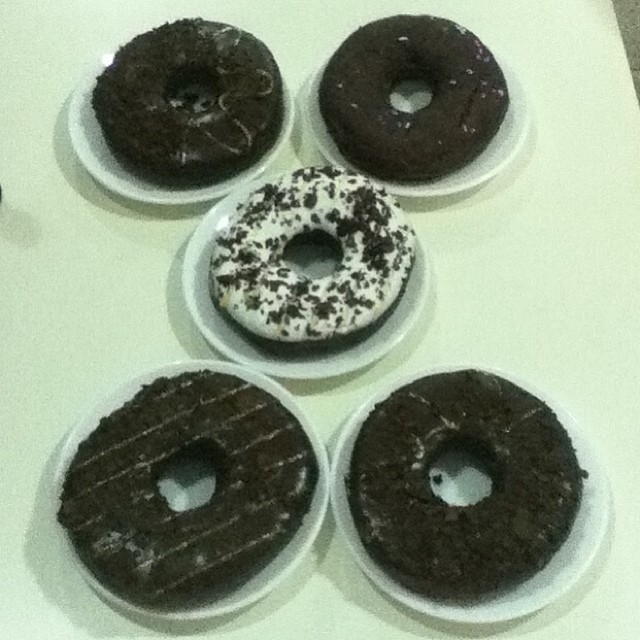This is an overhead photograph of a table featuring five round, white disposable plates, each holding a single doughnut. The table surface is smooth and white, not covered by a tablecloth, as evidenced by the visible edge at the corner of the image. The arrangement of the plates forms an X-like pattern, with two plates at the top, one centrally below them, and two more below the central one. The doughnuts, which are larger than typical in size, appear to be majority chocolate-based, characterized by a dark brown color. Among these, there is variation: one doughnut with white spots, another with white squiggles, one plain, and one with white stripes. The central doughnut stands out with its white frosting and crumbled cookie pieces on top. The photograph might be in black and white or very low color, making the dark doughnuts particularly prominent against the white plates. The doughnuts also have heart-shaped cutouts in the center, adding to their visually appealing presentation. These appetizing treats, with their different decorations, create a visually satisfying composition.